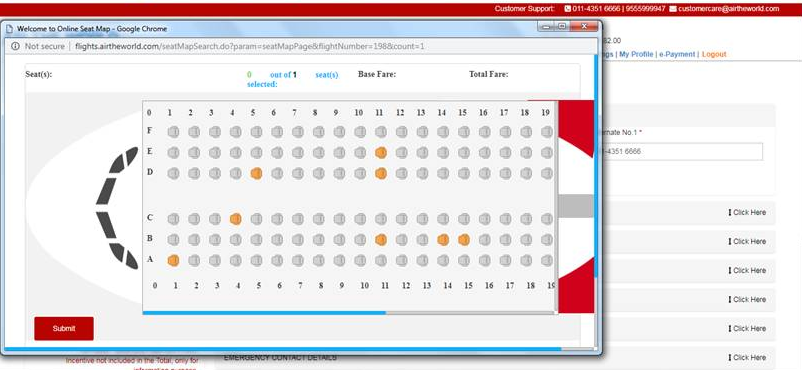The image is a screenshot of a website displaying a seating chart for flights. The background color is predominantly white. At the very top, there is a red border with "Customer Support" written in a white font on the right side, alongside a phone number and an email address, both also in white.

On the upper left corner, there is a rectangular dialog box outlined in sky blue. Within this box, in a gray font, it says, "Welcome to Online Seat Map." The webpage's address, "flights.airoftheworld.com," is visible, indicating that this is an online flight booking platform.

The main focus of the screen is the seating chart, which has a white background. The rows are numbered, and the seats are represented by simple gray icons; a few seats are highlighted in yellow. At the very top of the chart, it says "Seats," followed by "Out of One," "Base Fare," and "Total Fare." No actual pricing or numerical details are displayed in this section.

In the lower-left corner of the image, there is a red rectangle with the word "Submit" written in white, likely used for finalizing the seat selection.